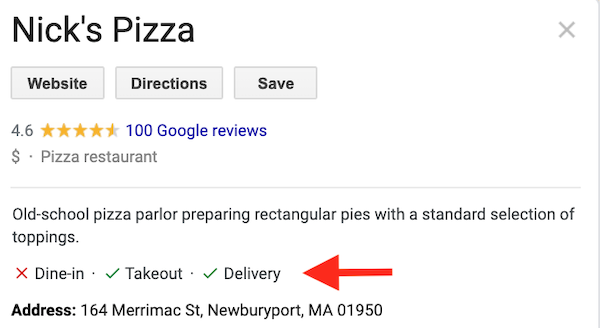This is a detailed image description of a screenshot of a Google search result for a restaurant named Nick's Pizza. The search result displays several interactive tabs including "Website," "Directions," and "Save." The restaurant boasts a rating of 4.6 stars out of 5, based on 100 Google reviews. It is categorized as inexpensive and is identified as a pizza restaurant. The description highlights that Nick's Pizza is an "old-school pizza parlor" known for preparing rectangular pies with a standard selection of toppings. It is noted that the restaurant does not offer dine-in options, but provides takeout and delivery services. A prominent red arrow points to the delivery option, emphasizing its importance. The address is listed as 164 Merrimack Street, Newburyport, Massachusetts, 01950. At the top right corner of the screenshot, an "X" icon is visible, allowing users to exit the search result. The size and prominence of the arrow pointing to delivery indicate a particular focus on this service within the displayed information.